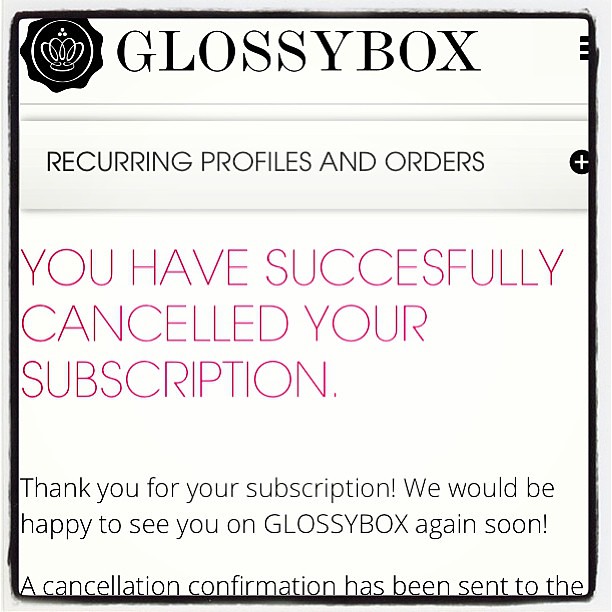The image is a cancellation notice from Glossybox, seemingly designed to resemble a letter sent through the mail rather than an email. It features a black border framing a white background. At the top, there is the Glossybox logo: a circular black emblem containing a white circle with a crown silhouette. The text "Glossybox" appears prominently in black, followed by "Recurring Profiles and Orders" in smaller print. Central to the image, in bright pink letters, it states, "You have successfully cancelled your subscription." Below this message, in black text, it reads, "Thank you for your subscription. We would be happy to see you on Glossybox again soon!" The notice concludes with the phrase, "A cancellation confirmation has been sent to the..." with the rest of the sentence cut off by the image's border. The notice is easy to read with no frills, suggesting a straightforward and customer-friendly business approach.